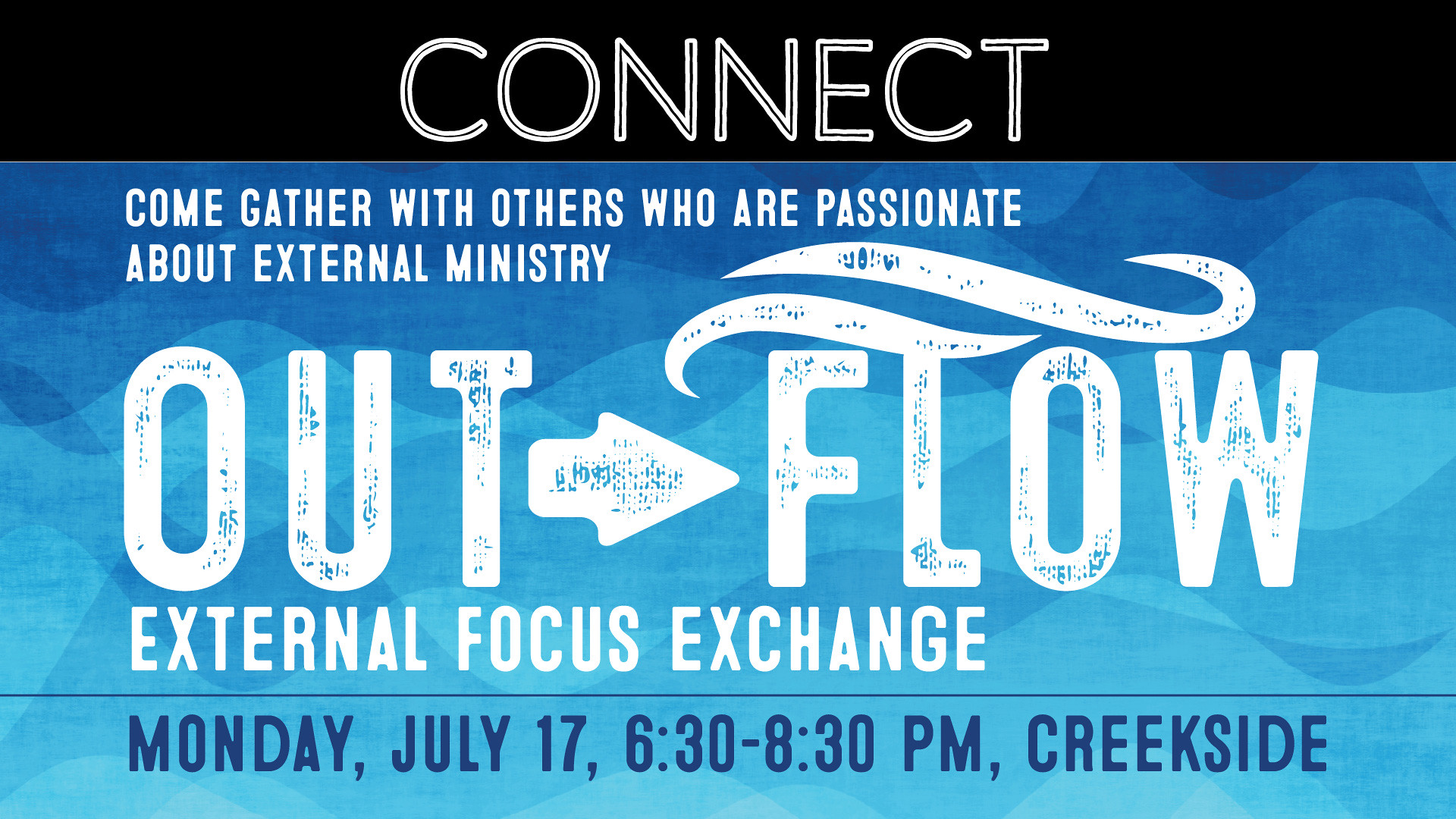This visually striking event poster predominantly features a blue background with a wavy motif, transitioning from darker to lighter shades to resemble ocean waves. A solid black rectangular section spans the top fifth of the poster, housing the prominent white block letters spelling "CONNECT." Below this section, in smaller white text, the message reads, "Come gather with others who are passionate about external ministry."

Centrally positioned on the poster, large, bold white letters spell "OUT," accompanied by a right-pointing arrow leading to the word "FLOW." Following this, the text "EXTERNAL FOCUS EXCHANGE" is presented in all-capital white letters.

Toward the bottom, a thin horizontal dark blue line divides the content, beneath which the event details are given in dark blue lettering: “Monday, July 17th, 6:30 to 8:30 p.m., Creekside.” This thorough and cohesive design effectively conveys information about an engaging workshop or event.